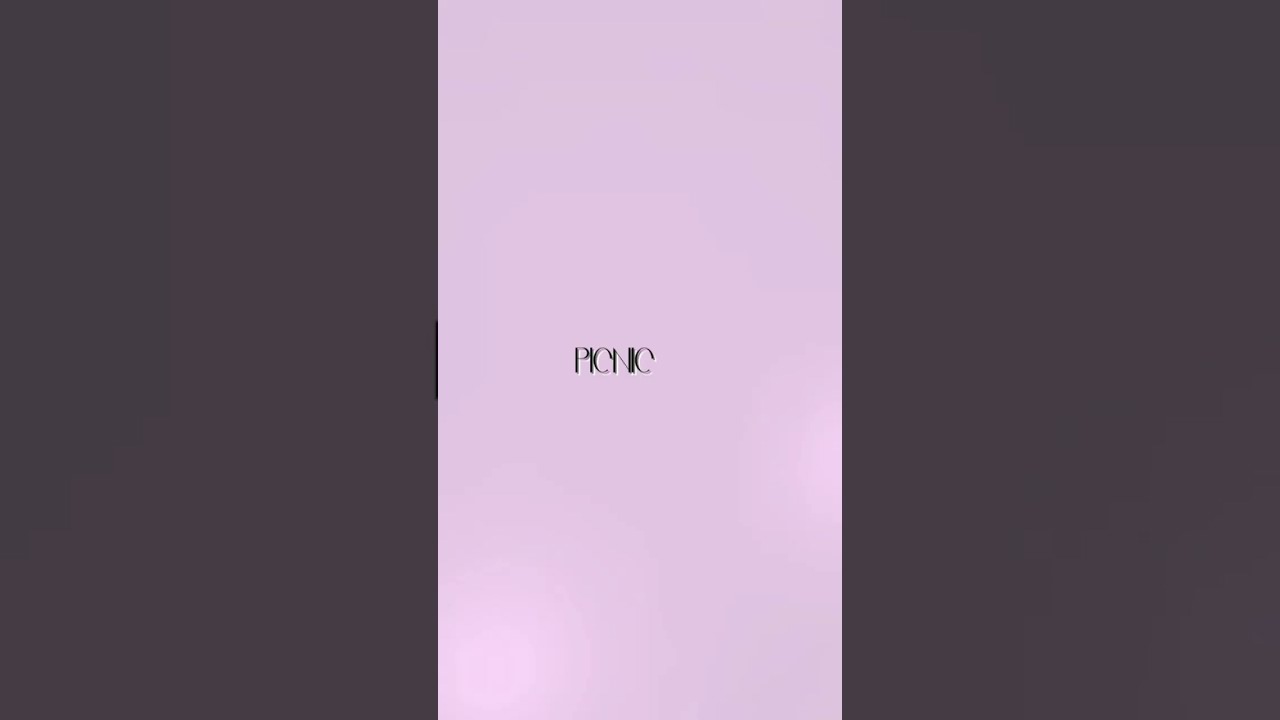The image is a simple, vertically oriented rectangular design. It features a central light pink stripe running from the top to the bottom of the frame. Positioned slightly to the left and below the middle of this pink stripe is black text in all capital letters that spells out "PICNIC." The letters are extremely close together, with the "I"s almost completely merging with the surrounding characters. On either side of the pink stripe are dark gray strips, each occupying about one-third of the image's total width. This image could be reminiscent of a minimalist advertisement, book cover, or movie poster with a clean and modern aesthetic. The overall composition, with its contrasting colors and central focus on the word "PICNIC," creates a striking yet simple visual.